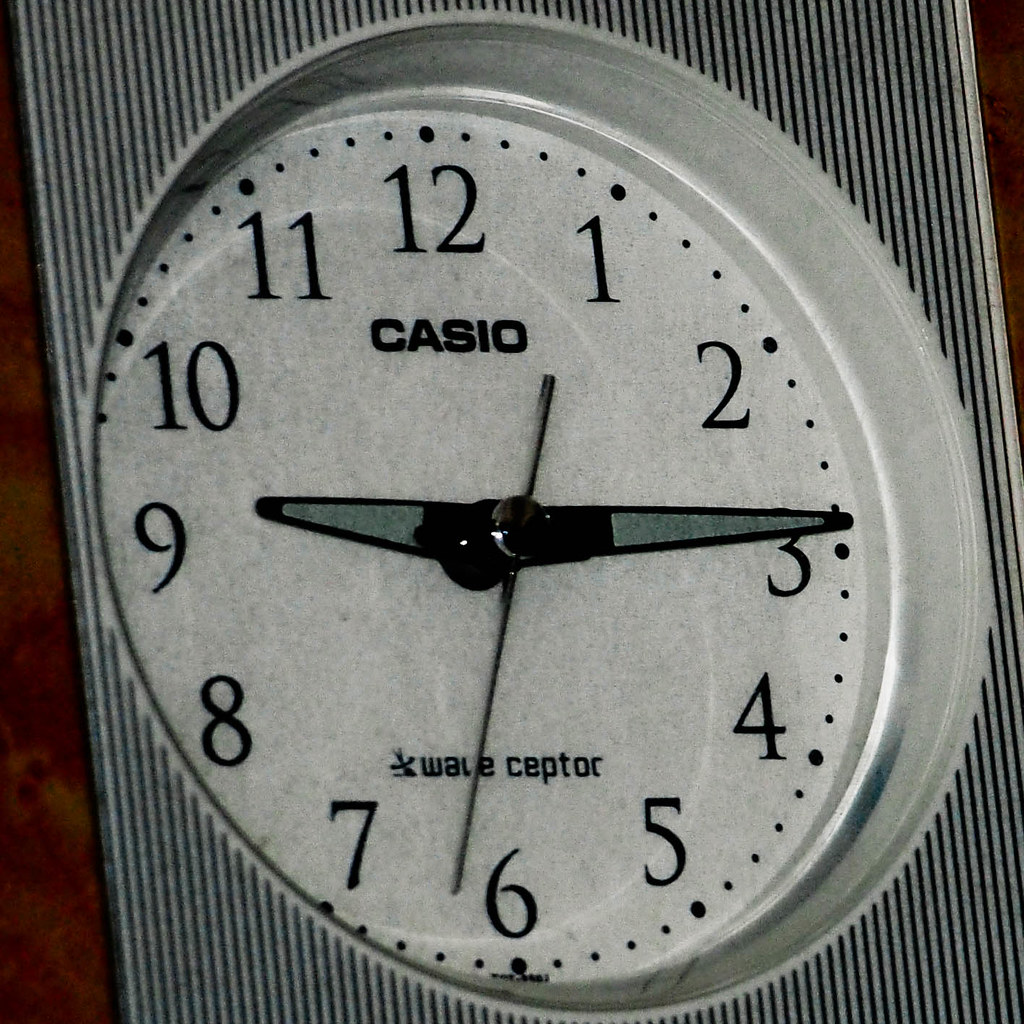This close-up photo captures an analog clock with a meticulously detailed design. The clock face is circular and set into a metal casing, which takes a rectangular shape. The exterior of the rectangular casing is adorned with thin, vertical pinstripe lines, adding an elegant touch to the clock. The brand name "Casio" is prominently displayed just below the 12 o'clock marker, while the term "Wave Ceptor" and a small cross logo are positioned above the 6 o'clock marker.

The hour and minute hands are long triangular shapes, accented with smaller grayish-green inset triangles. The slender second hand is a striking black, contrasting the other hands. Around the face, large, Roman numeral-style numbers from 1 to 12 are evenly spaced, each accompanied by a dot to mark the hour. Smaller black dots fill the spaces between larger hour dots to indicate minute and second intervals with precision. The overall composition exudes a blend of modern functionality and classic design elements.